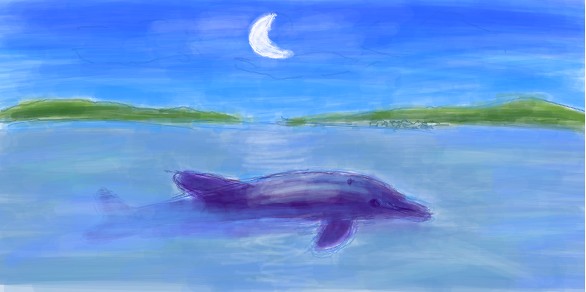The image is a colorful and somewhat simple illustration done primarily in markers or watercolor. It depicts a dolphin swimming in the ocean, with only its top half, including its fin, back, and face, visible above the water's surface. The dolphin itself is a darker blue, contrasting with the lighter blue hues of the water through which horizontal streaks run. The dolphin's lower body can be seen beneath the water’s surface. 

This rectangular, landscape-format artwork shows a distant line of green land formations on the horizon, possibly islands, which split the sea and sky near the top edge of the image. Above this land, the sky is nearly the same blue as the water with subtle, white striations suggesting clouds or mist. At the center of the sky is a white crescent moon, adding a celestial element to the serene scene.